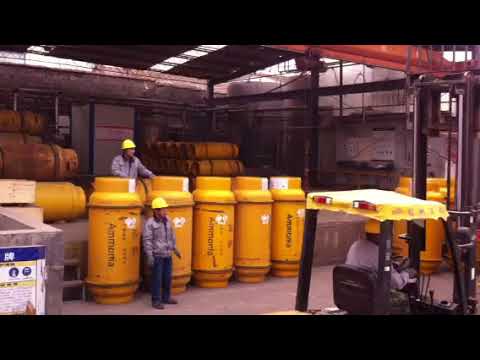This image depicts an industrial storage area within a warehouse setting. The floor is constructed from concrete and the space features a tin roof colored red. The environment is well-lit, with the ceiling supporting visible lights. Dominating the scene are numerous yellow-orange cylindrical containers, each marked with black writing indicating "ammonia." These containers are arranged in a row that spans the center of the image and are as tall, if not taller, than the workers standing before them.

In the foreground, a lifting vehicle or forklift is visible, partially entering from the right side of the frame. The forklift has a yellow roof and a black seat, occupied by a worker wearing a yellow hard hat, similar to the other workers present. Among the workers, one wears a gray long-sleeved jacket and blue jeans, standing directly in front of the containers, while another can be seen in the background dressed similarly.

Additional cylindrical containers are also visible laying horizontally on an elevated platform in the background, suggesting organized storage practices. The scene is clutter-free, emphasizing the predominant colors of yellow, gray, red, black, and blue within the setting. There are no texts apart from the labels on the containers. The photograph is internally framed with horizontal black bars at the top and bottom, providing a stark boundary to the industrial scene.